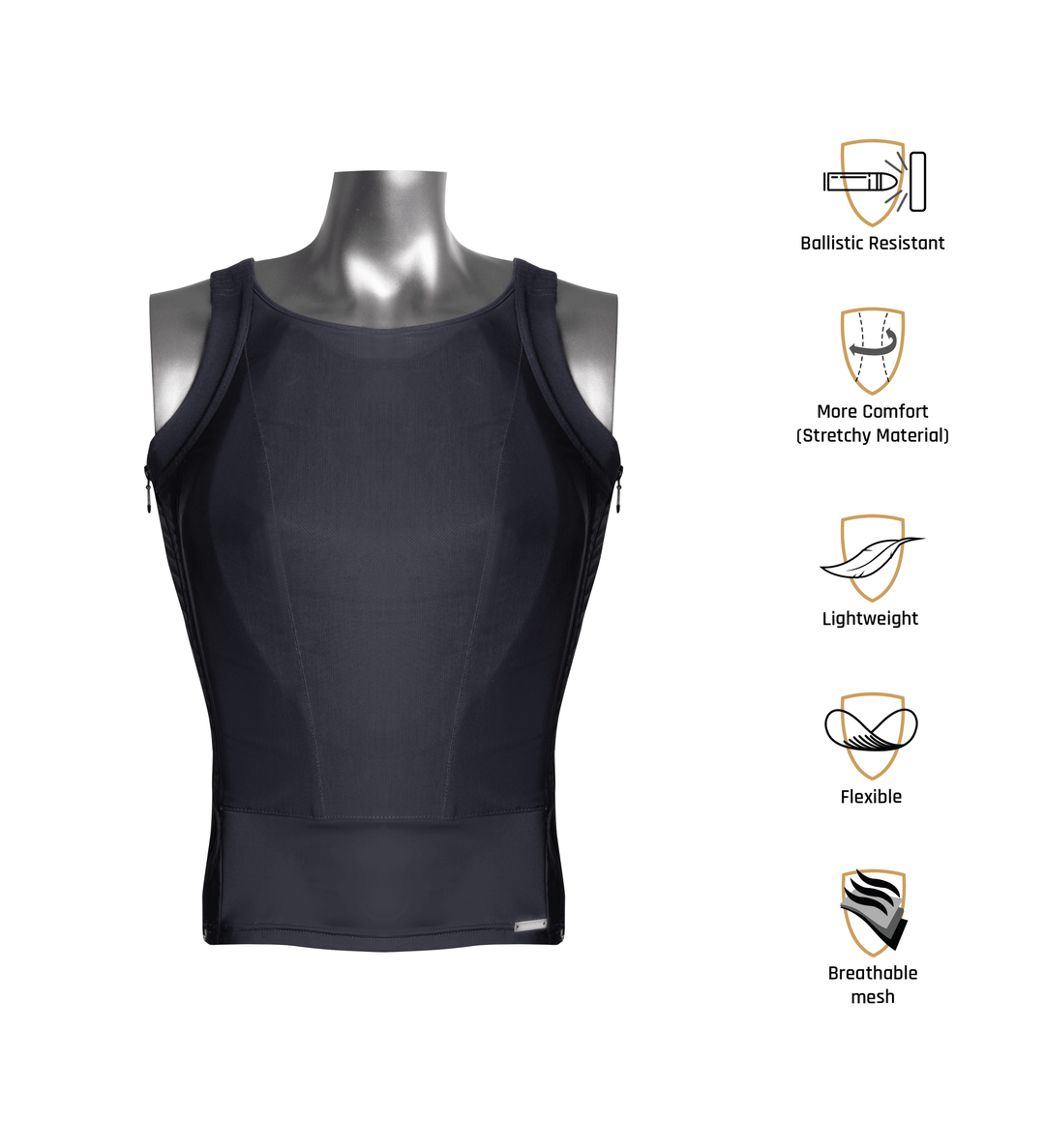The advertisement features a silver, headless and armless mannequin on the left side, set against a stark white background. The mannequin is styled as an athletic female torso and is dressed in a form-fitting, sleeveless dark blue tank top made from an elastic material. On the right side of the image, there are five yellow shield icons, each paired with descriptive text. 

Starting from the top, the first shield displays a bullet, labeled "Ballistic Resistant." The second shield, with an arrow encircling it, is labeled "More Comfort" with a note on stretchy material. The third shield features a feather, denoted as "Lightweight." The fourth shows two interconnected hoops and is marked "Flexible." The fifth and final shield contains an image suggesting heat waves and is captioned "Breathable Mesh."